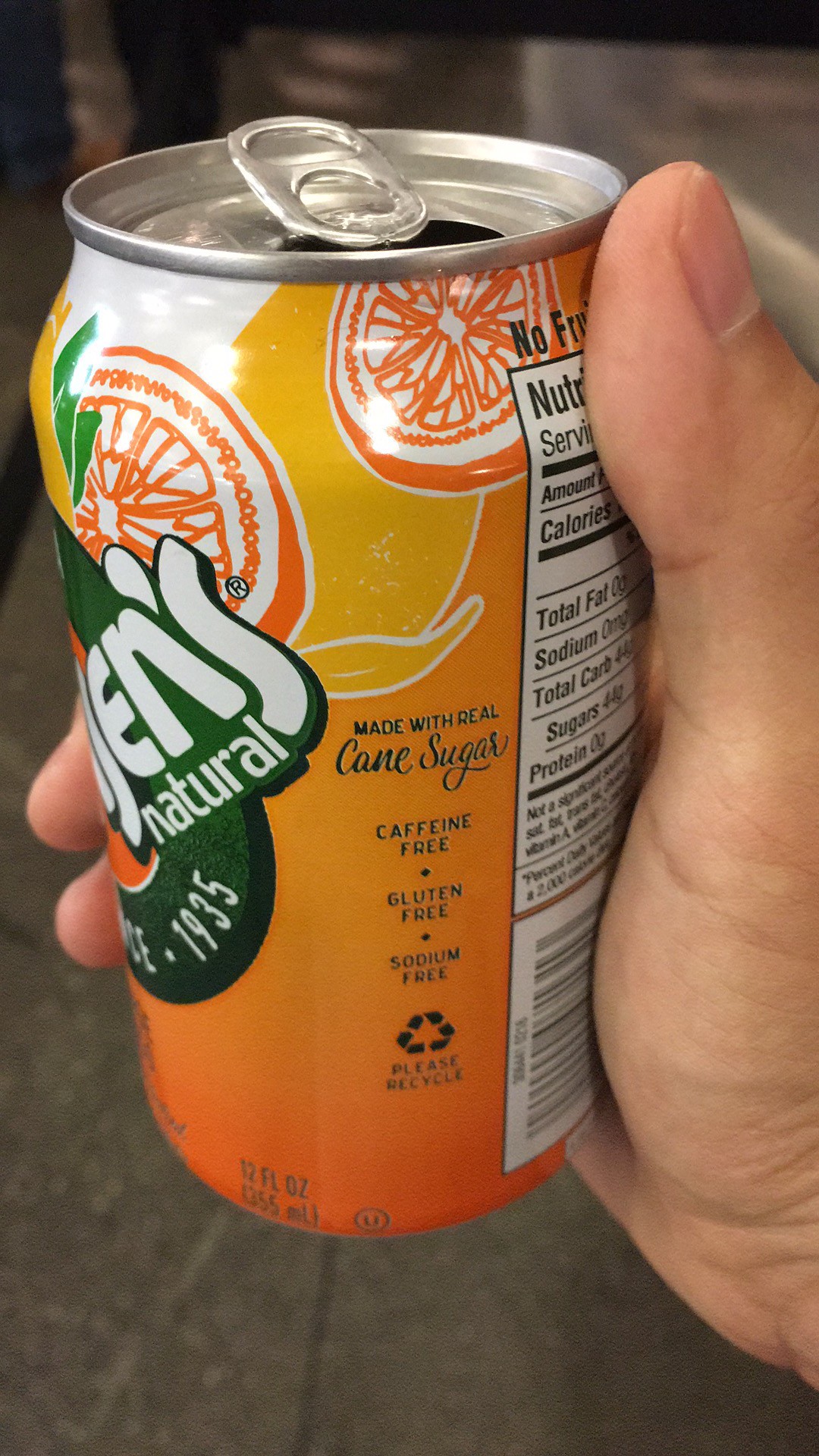The image is a vertical photograph showcasing a person's right hand holding an open aluminum soda can. The thumb and several fingers are visible, gripping the can with the thumb facing up and the palm inward. The can, predominantly orange with yellow accents, features graphics of orange slices and leaves. A green circular label on the can reads "JEN's natural 1935." The soda can is also marked with "made with real cane sugar," "caffeine-free," "gluten-free," "sodium-free," and "please recycle," along with nutritional facts partially visible on the side. The can is labeled as containing 12 fluid ounces or 355 milliliters. The background of the image is a dark gray and black color.